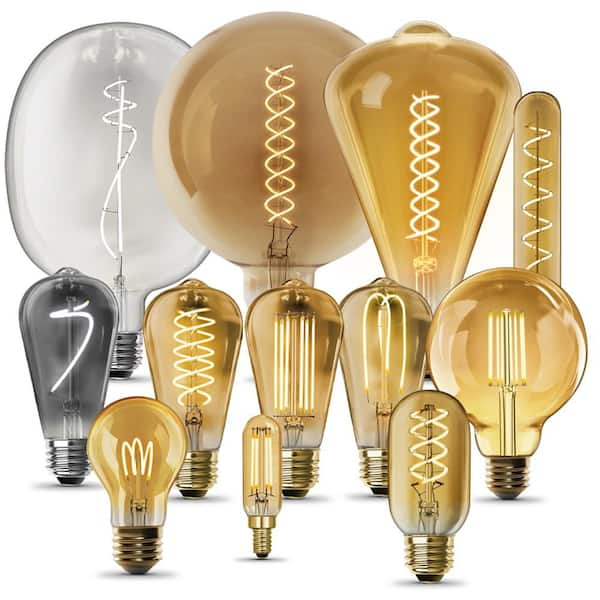The image features a collection of 12 distinctive light bulbs, each illuminated to reveal the intricate designs within. These bulbs vary greatly in size and shape, ranging from small to very large, and exhibit a diverse array of forms including circular, oval, conical, and tubular. Most of the bulbs are transparent, showcasing the artistic and deliberately designed filaments inside, which create unique patterns such as spirals, vertical lines, and double helixes. The glowing wires within the bulbs produce a range of colors from yellowish and golden to clear, white, and even grayish-black. The majority of the bulbs possess a yellowish tint with intricately arranged filament designs, giving them a vintage, almost hipster appeal. The light emitted by the bulbs enhances their aesthetic, making the intricate filament patterns and various shapes stand out beautifully.